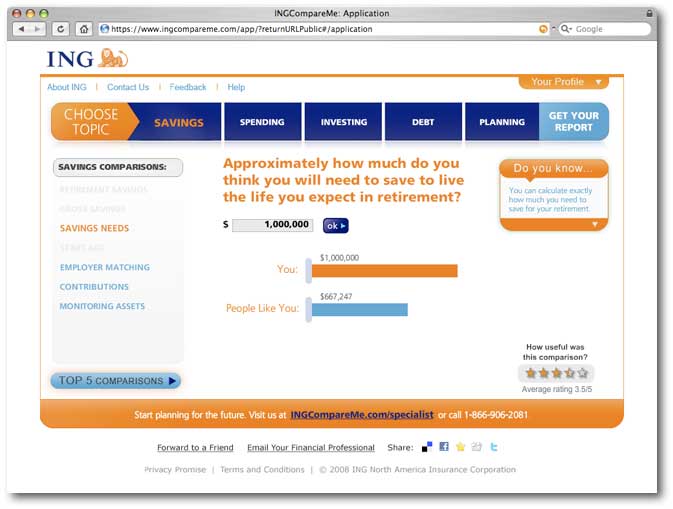The image depicts a webpage from INGCompareMe.com, viewed in Safari on macOS. Positioned prominently at the top left is the distinctive ING logo, featuring a golden lion statue seated regally. The navigation bar at the top includes essential links: "About ING," "Contact Us," "Feedback," and "Help." To the right of these links is a profile section with a dropdown menu for additional options.

The main content area of the page presents a series of topics users can explore, such as "Savings," "Spending," "Investing," "Debt," "Planning," and "Get Your Report." Below this is a prompt asking, "Approximately how much do you think you will need to save to live the life you expect in retirement?" A user has entered $1,000,000 and clicked "Okay." The results are displayed with two bars: one labeled "You" with the entered amount of $1,000,000, and another labeled "People like you" with a suggested amount of $667,000, indicating a potential overestimation by the user.

On the left side of the page are additional links related to saving strategies, such as "Saving Needs," "Employer Matching," "Contributions," and "Monitoring Assets." A contact phone number is conveniently located in the bottom right corner for further assistance.